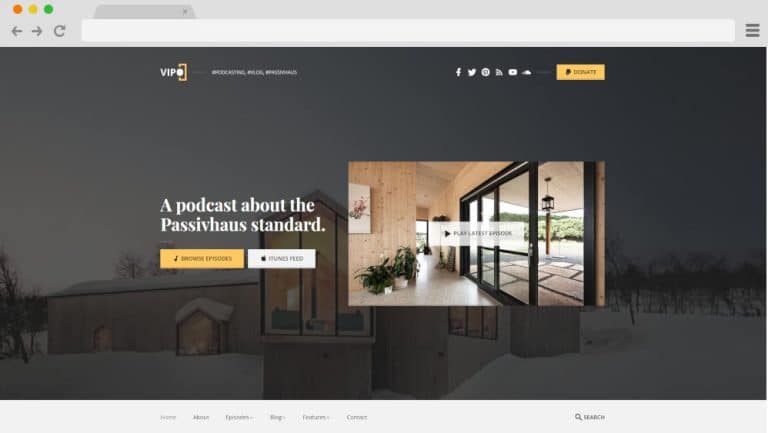This image showcases a detailed website mock-up featuring a sophisticated and modern design. The background is predominantly grey. At the top, there's a blank tab followed by an integrated search bar. Below this header, the central content begins with an image banner displaying a sleek, modern house with large windows, surrounded by snow. The image is layered with a semi-transparent dark filter, enhancing the bold white text overlay on the left that reads "A Podcast about the Passive House Standard."

Beneath the text, there are two call-to-action buttons: an orange button labeled "Browse Episodes" and a white button labeled "The Feed." To the right of this section is a striking large thumbnail depicting the modern interior of a house. Central to this thumbnail is another semi-transparent white bar with the text "Play Latest Episode."

The bottom section of the mock-up maintains the grey theme and features six distinct category listings, providing easy navigation options. At the far right of the bottom section is a search icon, facilitating user convenience in exploring the website further.